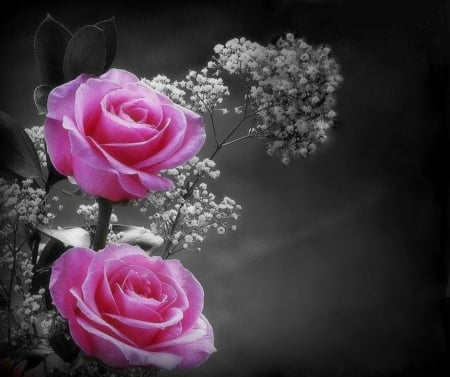This photograph features a vivid contrast between two vibrant pink roses and a grayscale background, creating a dramatic and serene composition. The roses, brightly lit and displaying a delicate gradient from hot pink to soft pink, are the focal point and the only elements in color. Arranged one atop the other, they are fully blossomed, with intricate petals illuminated by soft lighting. Behind and around the roses are soft, white baby's breath flowers and a few eucalyptus leaves, blending into the grayscale background. The background itself transitions from a lighter gray behind the flowers to a darker, almost black shade towards the corners, particularly the upper right. The image, professional and photorealistic, except for its artistic color alteration, positions the floral arrangement mostly on the left side, extending slightly past the center. The dramatic use of black and white accentuates the vibrancy of the pink roses, making them the undeniable centerpiece of this serene, almost postcard-like photograph.